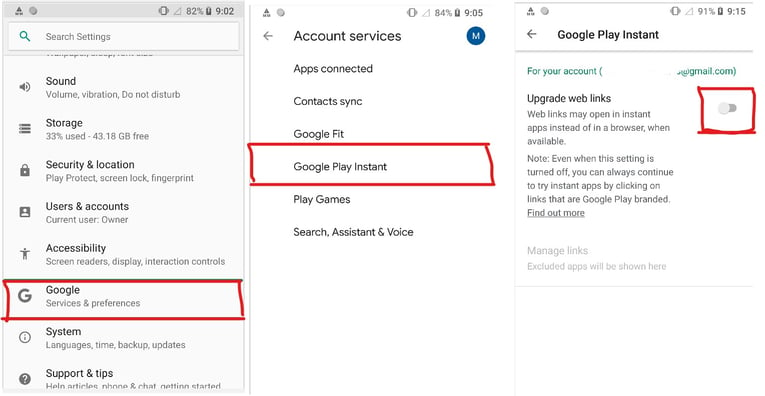This is a series of three sequential cell phone screenshots, displayed side by side, forming a step-by-step tutorial. 

The first screenshot is from a settings panel. At the top, there is a search bar labeled "Search settings." Below the search bar, various categories are listed, including Sound, Storage, Security & Location, User & Accounts, Accessibility, and Google. The 'Google' category is highlighted with a red box, indicating it is the next step.

The second screenshot zooms in on the 'Account services' section. Several options are listed vertically: Apps Connected, Contact Sync, Google Fit, and Google Play Instant. The 'Google Play Instant' category is highlighted with a red box, guiding the user to the next step.

The third screenshot focuses on the 'Google Play Instant' settings. Below the heading "For your account," the user's email has been blurred for privacy. Underneath, there is an option labeled "Upgrade web links," accompanied by a toggle switch on the right side. This switch, which is currently in the off position, is also highlighted with a red box for emphasis.

Together, these screenshots create a clear and detailed tutorial on navigating through various settings to find and manage the "Upgrade web links" toggle under 'Google Play Instant.'